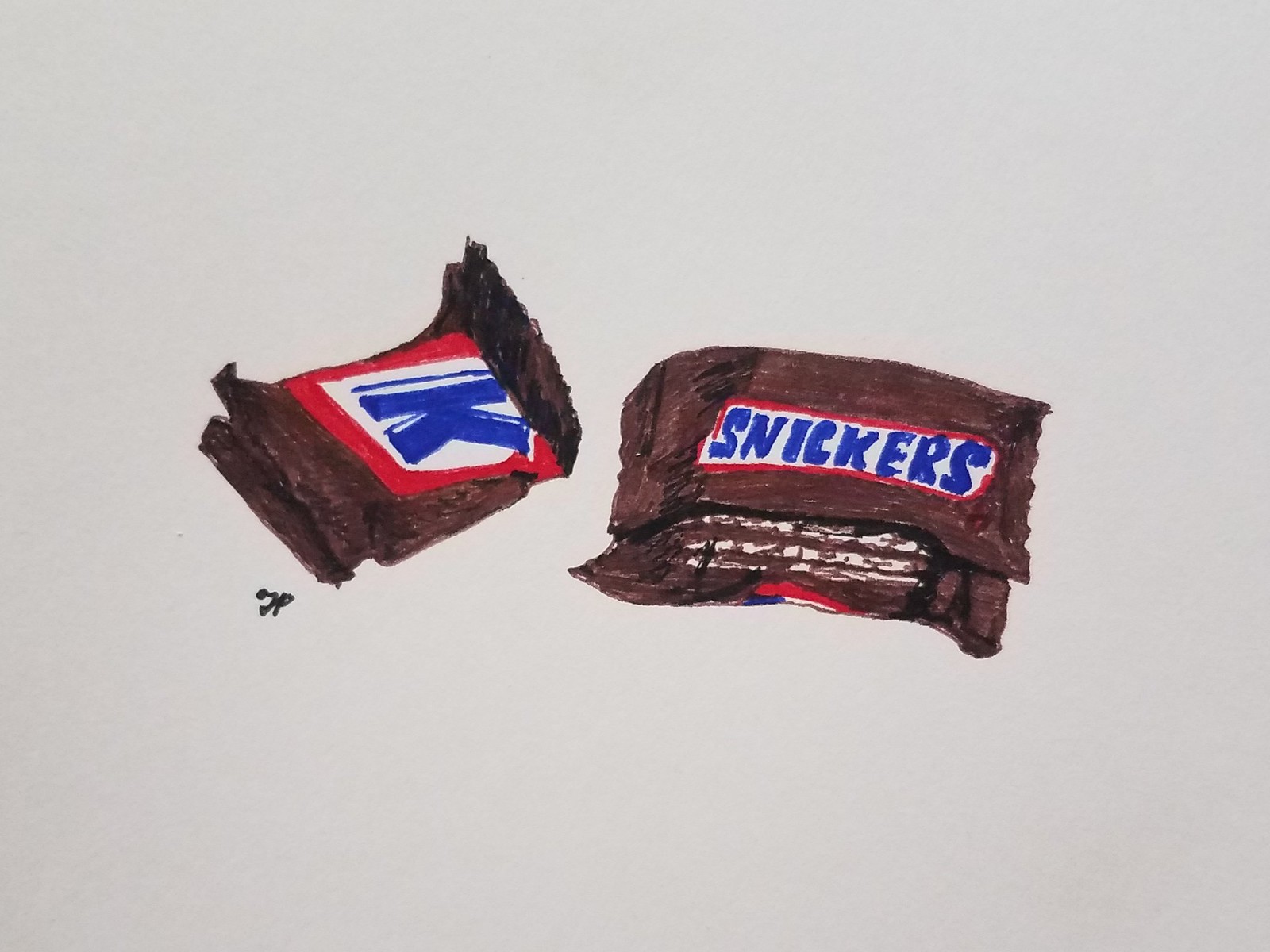This image appears to be a detailed drawing or painting of Snickers mini candy bar wrappers set against a grayish-blue background. On the right side, there is a depiction of a Snickers wrapper. It features the typical brown wrapper, with the word "Snickers" prominently displayed in large blue letters on a white background, surrounded by a red outline. The wrapper seems slightly ambiguous as to whether it contains the candy bar or not. 

To the left, there's another depiction of a Snickers wrapper, which appears to be folded multiple times. The folded wrapper also has a brown color, with a red frame and a white background, showcasing a large blue letter "K." It's more angled compared to the more straight depiction on the right. Intriguingly, the left-side section includes what seem to be small initials "KP," likely representing the artist's signature. Throughout the image, the detailed rendering captures the iconic branding of Snickers in red, white, and blue against a brown wrapper, symbolizing the familiar and beloved treat in its mini form.